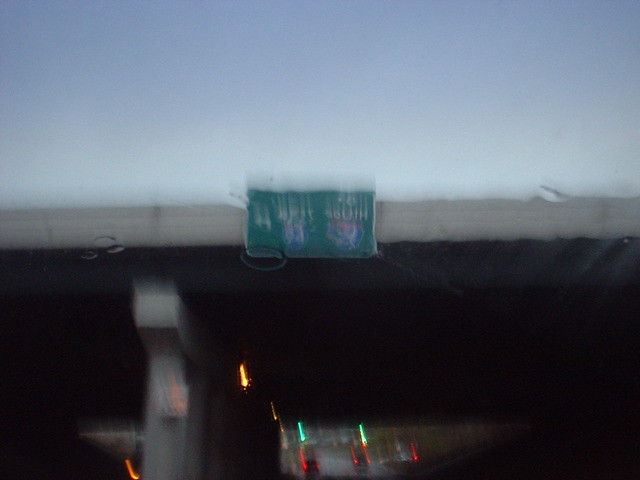The photograph, taken from inside a moving car, captures a rainy day scene on a busy highway. The image features a blurry overpass stretching horizontally from left to right, supported by large concrete pillars positioned just left of center. A nearly unreadable large green rectangular sign is attached to the overpass, displaying highway directions with visible indication of Interstate 94 and a directional arrow. The scene in the foreground is marked by raindrops on the windshield, while the bottom portion of the image shows the distant brake lights of cars. Despite the overcast conditions, a patch of blue sky peeks through, creating a contrast above the darkened area under the overpass.